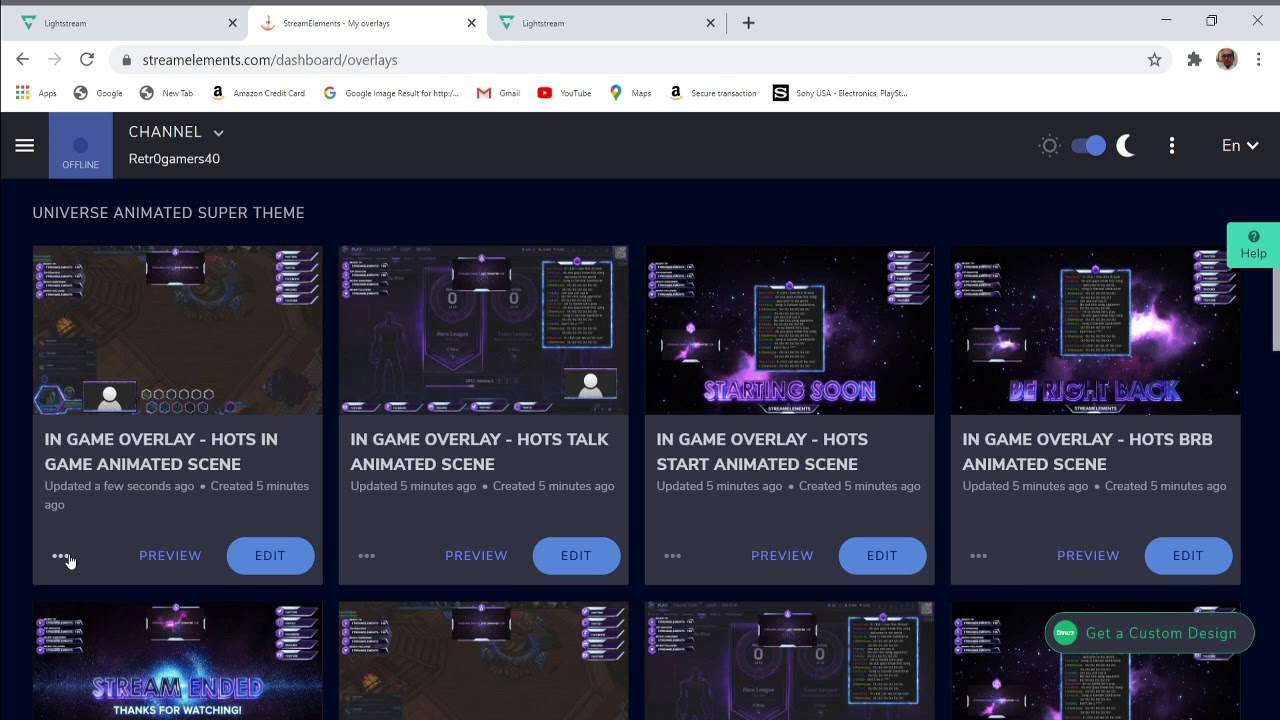The image displays the home page of a YouTube channel, viewed on a desktop device using the Microsoft Edge browser with a gaming overlay. The interface is set to night mode, as indicated by the dark theme and the moon icon toggled on the right side of the screen. The page showcases an animated in-game scene, with the same title repeated across four thumbnails, although only the top halves of the bottom row of thumbnails are visible. The interface also shows the three-dot menu (indicating additional settings) and a language mode drop-down menu labeled "EN." The overall layout and features signify a YouTube channel customized with night mode for a darker, more visually comfortable viewing experience.